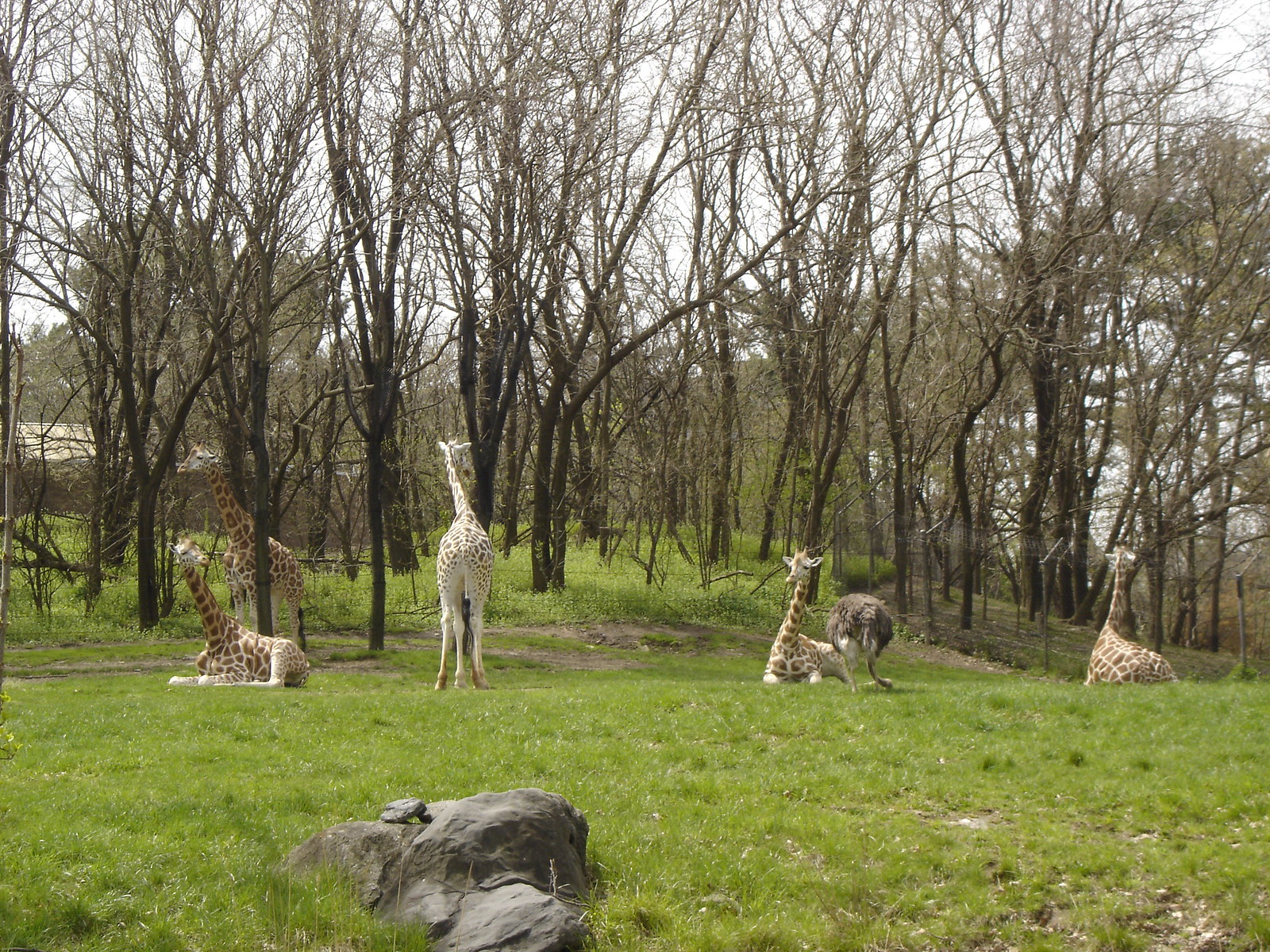In a serene wildlife preserve, a wide, lush green field stretches out, dotted with six majestic giraffes. Three of these towering creatures are peacefully lying down, curled up with their necks gracefully outstretched. The giraffe second from the left stands out with its lighter, predominantly white coloration, standing tall amidst the sparse, budding spring foliage. To the right, another giraffe stands with its back towards the observer, showcasing its distinctive spots.

In the distance, thin woods just beginning to sprout new leaves blend with a backdrop of fully-leaved trees, and a building peeks through this tranquil scene, suggesting a facility dedicated to the care of these magnificent animals. To the right of the meadow, near the resting giraffes, a rounded figure with gray feathers and a white underside—it appears to be an ostrich—leans down, almost blending into the peaceful tableau. A large, gray boulder juts out from the bottom left of the field, adding a natural touch to the landscape.

Overall, the image captures a moment of tranquility in a preserve where giraffes and an ostrich coexist harmoniously among the spring green grass and budding trees.